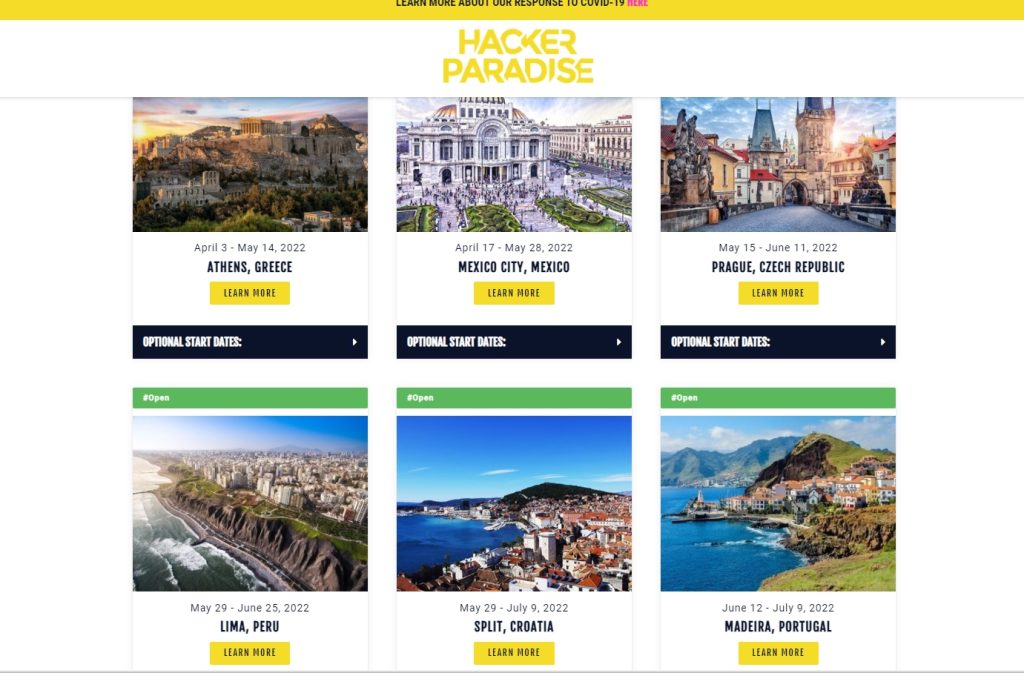This image is a detailed screenshot of a web page. 

At the very top, there is a prominent yellow bar with black text that reads, "Learn more about our response to COVID-19." Below this bar, the background shifts to white, and centrally positioned in striking yellow lettering is the phrase "Hacker Paradise."

The page layout then features two rows of destination options, each containing three locations.

In the first row:
1. On the far left is a section for Athens, Greece, which includes a scenic picture of Greece above the text that specifies the travel dates as April 3rd to May 14th, 2022. There is a yellow "Learn More" button and a black button to check optional start dates.
2. The middle section showcases Mexico City, Mexico. A vibrant picture of Mexico City appears above details about the destination, accompanied by the same yellow "Learn More" button and black optional start dates button.
3. On the far right is the segment for Prague, Czech Republic. Positioned above its text is a picturesque image of Prague, with the travel dates listed as May 15th to June 11th, 2022. Below this, there are the familiar yellow "Learn More" button and black optional start dates button.

In the second row:
1. On the far left is Lima, Peru. A beautiful picture of Peru is displayed, and the travel dates are from May 29th to June 25th, 2022. As with other destinations, there is a yellow "Learn More" button.
2. The center section is dedicated to Split, Croatia. It features a picturesque image of Croatia, with dates listed as from May 29th to July 9th, 2022, and includes the yellow "Learn More" button.
3. On the far right is Madeira, Portugal, which has a captivating image of Portugal above its text, with travel dates from June 2nd to July 9th, 2022, accompanied by the yellow "Learn More" button.

Each destination card provides a clear visual and textual representation, making it easy for users to explore more specific details and options for each location.